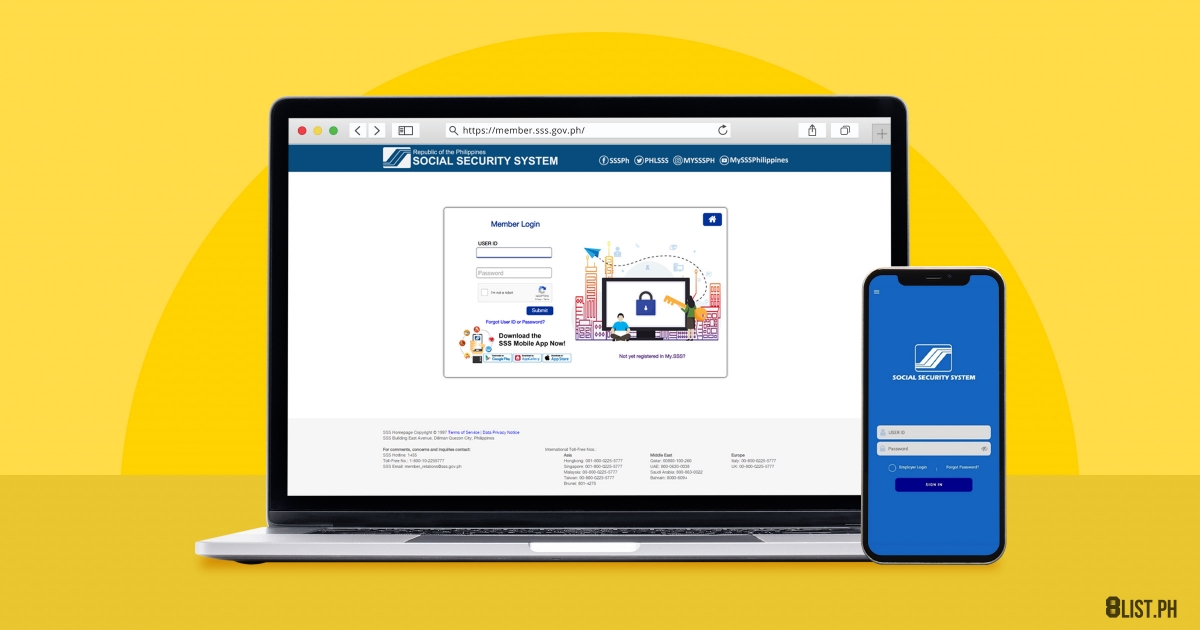The image depicts a promotional scene highlighting the Social Security System's online access points, featuring both a laptop and a smartphone displaying the organization's member portal. The laptop screen showcases the Social Security System’s homepage with a central focus on the member login section, presenting fields for user ID and password input, accompanied by an icon representing a user logging in. The layout includes a blue navigation bar at the top and a light gray footer at the bottom, with the main page content set against a white background.

Adjacent to the laptop, a smartphone displays the Social Security System’s mobile application login interface. The app screen features a solid blue background with two prominent gray text fields for entering the user ID and password, and a deep blue submission button for proceeding with the login. The image emphasizes the accessibility and consistency of the Social Security System's online services across different devices.